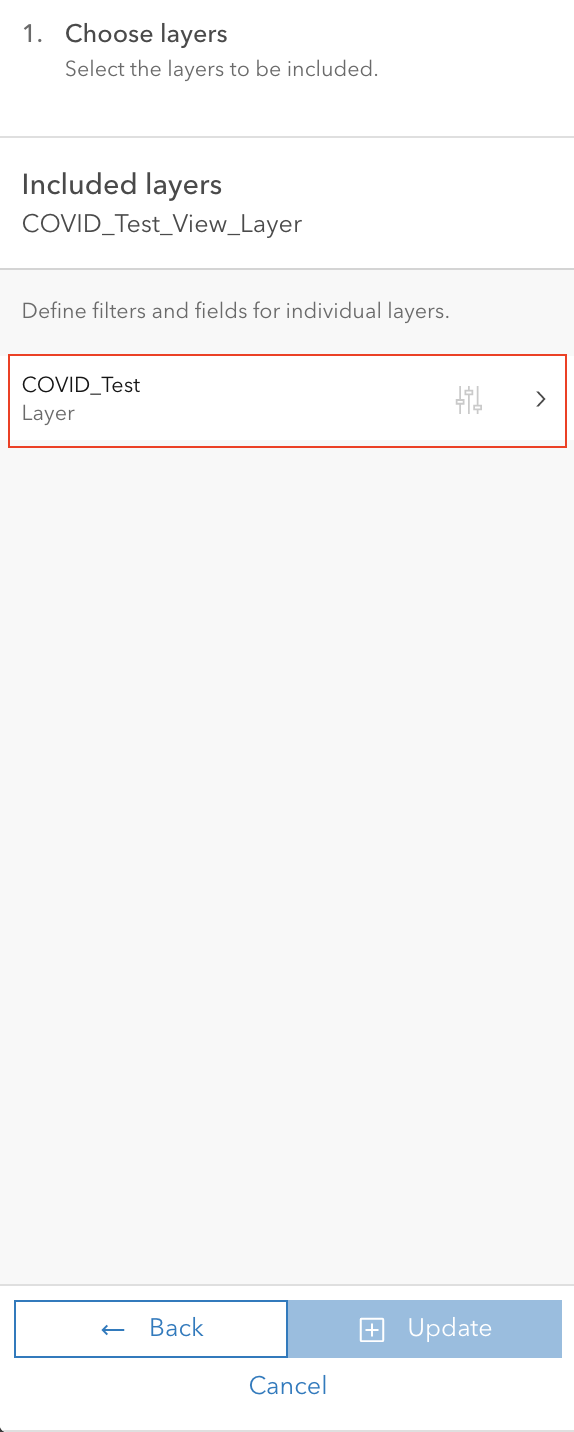This is a detailed caption for the screenshot:

---

The screenshot, taken on a cell phone, features a white background with black text outlining the following instructions: "1. Choose Layers," followed by "Select the layers to be included." Below this, a gray bar runs horizontally displaying "Included layers: COVID_test_view_layer." Beneath this bar, on a light gray background, the text reads "Define filters and fields for individual layers." Within this section, "COVID_test_layer" is highlighted with a red rectangle around it. To the right of this layer, standard filter icons commonly used in various apps are displayed, indicating options to filter this specific layer. Additionally, there is a right-facing arrow next to these icons, implying that clicking it will provide more information or allow changes to the filter settings. The rest of the page is blank until the bottom, where two interactive elements are present: a blue-outlined rectangle with white interior and blue text reading "Back" along with a left arrow, and to its right, a solid blue rectangle with white lettering that says "Update." Below these, the text "Cancel" appears in blue lettering.

---

This caption aims to offer a comprehensive description of the screenshot, detailing both visual elements and their functionality.